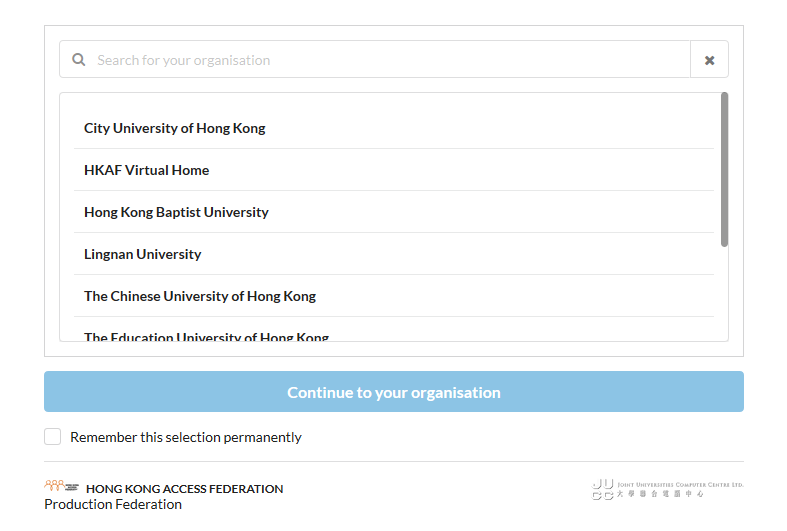The image displays a horizontally oriented white rectangle, likely representing a digital interface for the Hong Kong Access Federation (HKAF) and the Joint Universities Computer Center (JUCC), as indicated by the text in the bottom corners. In the bottom left corner, it states "Hong Kong Access Federation, Production Federation," while the bottom right corner reads "Joint Universities Computer Center, LTD," along with some Asian Kanji and the acronym "JUCC."

At the top of the rectangle, there is a search bar with the placeholder text "Search for your organization." Directly beneath this search bar, various organizations are listed in the following order:
1. City University of Hong Kong
2. HKAF Virtual Home
3. Hong Kong Baptist University
4. LINGNAN University
5. The Chinese University of Hong Kong
6. The Educational University of Hong Kong (partially cut off)

A gray scroll bar is present on the right side of the rectangle, suggesting the option to scroll and view more results. Positioned at the bottom of the rectangle is a wide, light blue button that spans the entire width of the rectangle, containing the text "Continue to your organization" in white. To the left of this button, there is a checkbox option labeled "Remember the selection permanently."